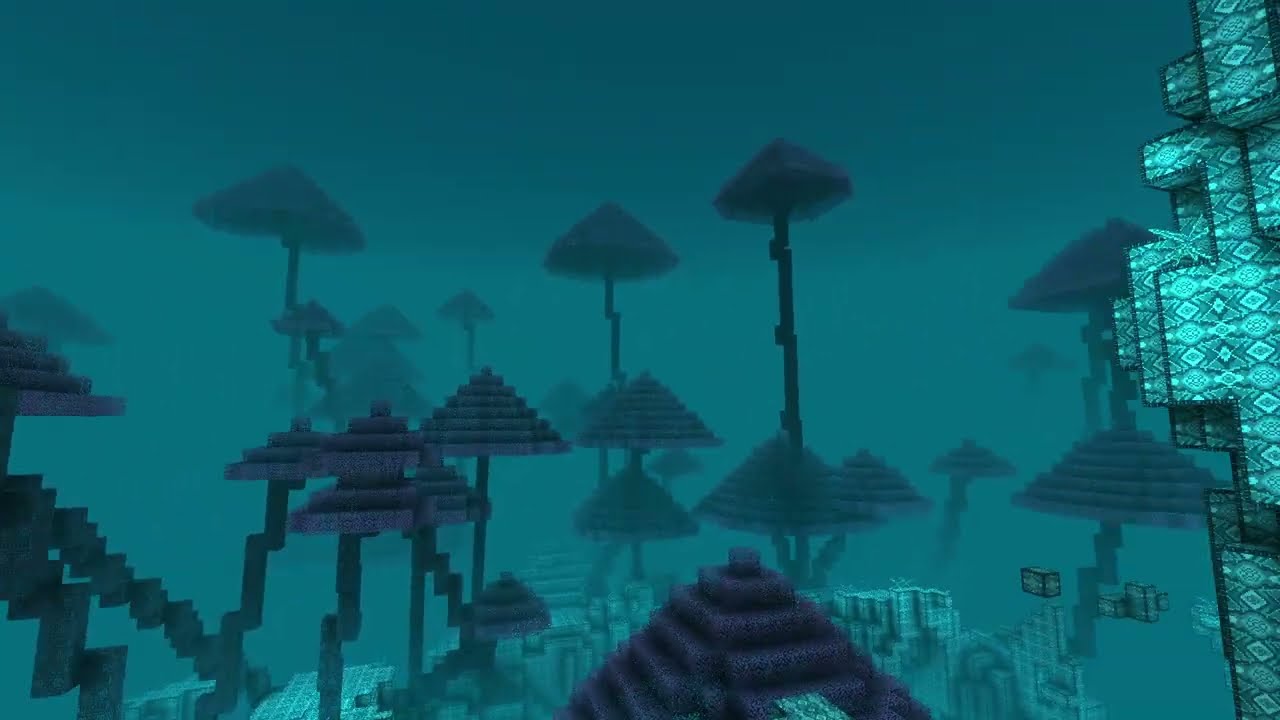The image features a detailed, pixelated landscape reminiscent of a video game, likely inspired by Minecraft. Set against a dark teal, underwater-like backdrop with a blue hazy fog, the scene showcases a multitude of structures resembling tree trunks or mushroom stems, each composed of jagged, blocky gray lines. Topping these stems are woven, umbrella-shaped canopies, pyramid-like and adorned with purple blocks that give them a layered appearance. Several of these prominent structures stretch horizontally across the middle of the image, with larger formations centrally located, and smaller ones appearing in groups toward the front and lower portions of the scene. Additionally, glass-like towers with circular teal patterns, resembling apartment buildings, rise along the right edge, adding to the complex, multi-dimensional digital environment.